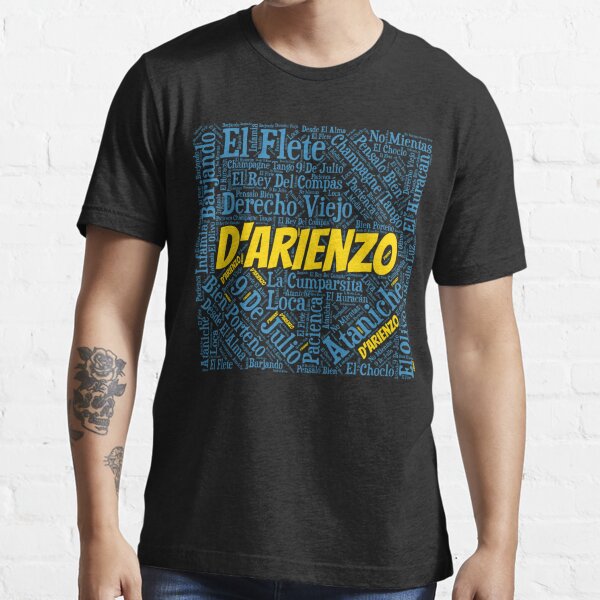The photograph shows a close-up of a white or Hispanic male wearing a black T-shirt, cropped just below his waist. His head is not visible in the image. The background features a solid, white painted brick wall. Central to the black T-shirt, in bold yellow capital letters, is the text "D-A-R-I-E-N-Z-O". Surrounding this are numerous blue words in Spanish like "derecho viejo," "el rey del compas," and "nueve de Julio," arranged vertically, horizontally, and diagonally. The man has tattoos on his right forearm, including one of a skull with a flower on its head, alongside another undecipherable tattoo near his wrist. His left arm does not have any visible tattoos. He is also wearing blue jeans. The composition and styling suggest this image is part of an advertisement for a clothing website.